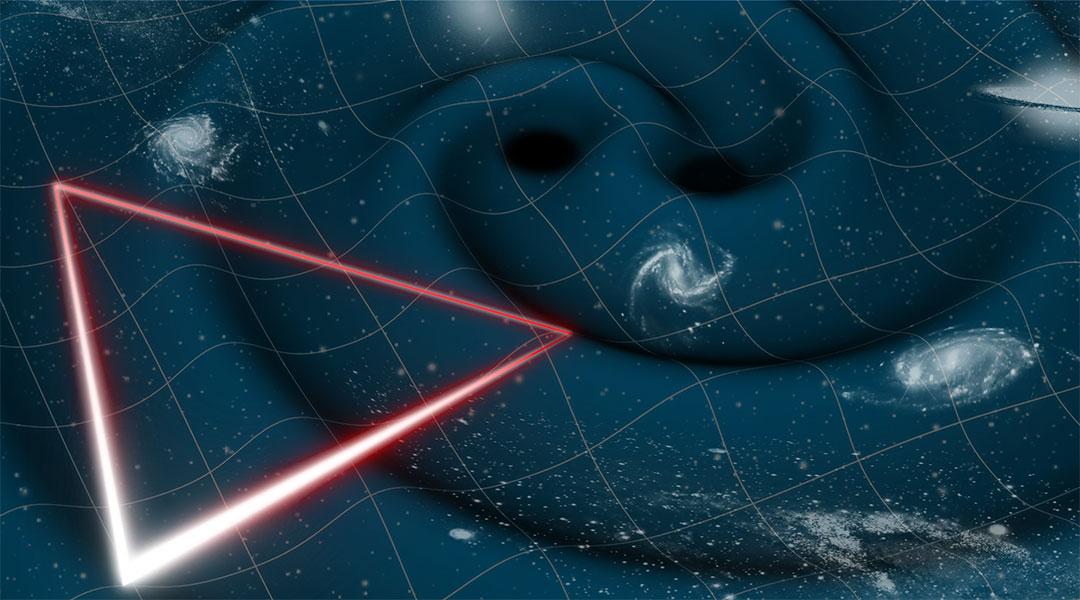The image is a horizontally oriented digital rendering, primarily dominated by a dark blue color scheme. The central focus is a fabric-like, contoured design that swirls in a spiral pattern, creating a wave-like texture. Towards the middle of this intricate swirl, there are two adjacent circular black spaces reminiscent of black holes. Scattered throughout the swirling dark blue are white stars and faint, galaxy-like formations, adding to the celestial theme. A delicate white grid overlays the entire design, bending and warping along with the fabric-like contours, enhancing the depth and movement of the space scene.

On the left side of the image, there is a prominent triangle composed of neon pink, red, and white light. This triangle is superimposed over the swirling pattern and is oriented such that its bright white bottom corner contrasts sharply against the dark background, while the top becomes a thin, almost indistinguishable red line. The overall effect of the image is a mesmerizing blend of a contoured space chart, interlaced with a dynamic fabric-like texture and striking geometric elements.